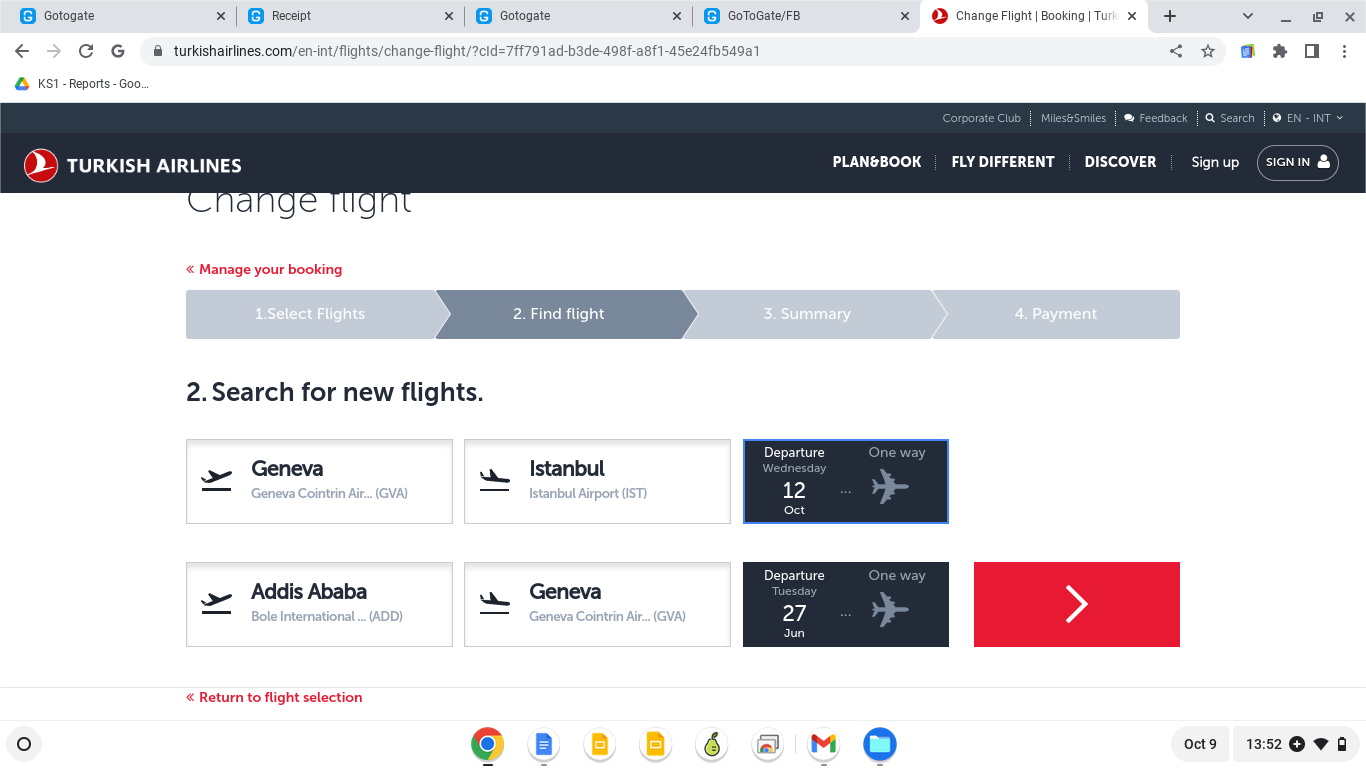The image captures a screenshot of a website dedicated to airline services. At the top left of the image, several browser tabs are open, five in total, with the current focus on the fifth tab. The first four tabs share a similar design, represented by a "G" logo set against a blue background, indicating they originate from the same website. They are labeled sequentially as follows: "Go to Gate," "Receipt," "Go to Gate," and "Go to Gate/FB." The fifth and currently active tab is titled "Change Flight."

Central to the image, prominently displayed on the website, is the Turkish Airlines brand. Positioned at the top left, the Turkish Airlines name is accompanied by its logo, featuring a white figure on a red circular background. On the far right side of the website's header are several navigation options: "Sign in," "Sign up," "Discover," "Fly Different," "Plan," and "Book," all rendered in white text.

Beneath the header, there is a section labeled "Change Flight," accompanied by four distinct steps: "Select Flights," "Find Flight," "Summary," and "Payment," each indicating a stage in the flight change process.